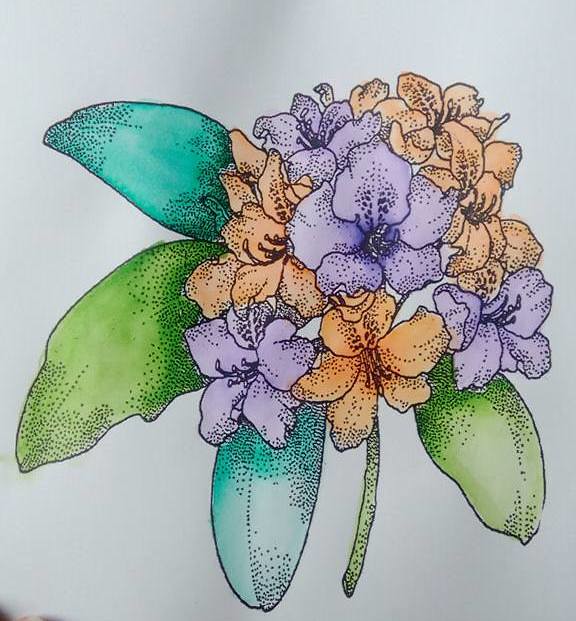This image features a vividly colored illustration, likely originating from a pre-drawn sketch commonly found in a coloring book. The artwork showcases an arrangement of flowers, each adorned with distinct petal designs. The first type of flower has petals that gracefully flow outward and downward, painted in a vibrant orange hue. The second type features flat, simpler petals, filled in with a rich purple color. Surrounding the flowers are four leaves, adding to the composition with their sharp, pointy shapes. Two of the leaves are a traditional green, while the remaining two sport a unique bluish-green tint, creating a harmonious blend of colors.